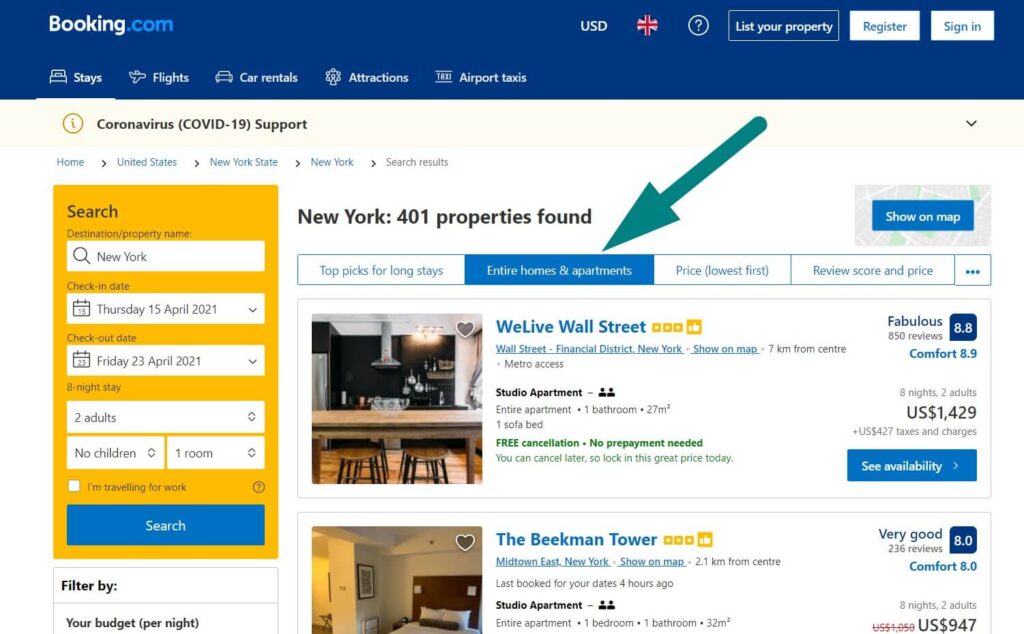This image is a screenshot from a website, featuring a dark blue background at the top with a white banner. In the top left corner, the text "Booking" is displayed; "Booking" is in white text with a capital "B," and ".com" is in blue text. Moving to the right, there is "USD" in white text accompanied by a burst flag, followed by a white circle with a white question mark inside. Further along, it says "List your property" with a white border around it, then "Register" and "Sign in."

Below this section, there is a navigation bar on a white background that includes the options: "Stays," "Flights," "Car rentals," "Attractions," and "Airport taxis." There is also a yellow circle with a white lowercase "i" inside, next to the text "Coronavirus (COVID-19) support."

Next, the breadcrumb trail reads: "Home > United States > New York State > New York > Search results." Below this, a yellow banner displays the search parameters: "Search: New York, Thursday, April 15, 2021 - Friday, April 23, 2021," indicating an eight-night stay for two adults, no children, in one room. It also includes another "Search" button.

Further down, there's a filter section titled "Filter by your budget per night," followed by details on the search results: "New York: 401 properties found." Additional filters and sorting options like "Top picks for long stays," "Homes and apartments," "Price goes first," "Review score and price," are listed. A jade arrow points to the option for "Entire homes and apartments."